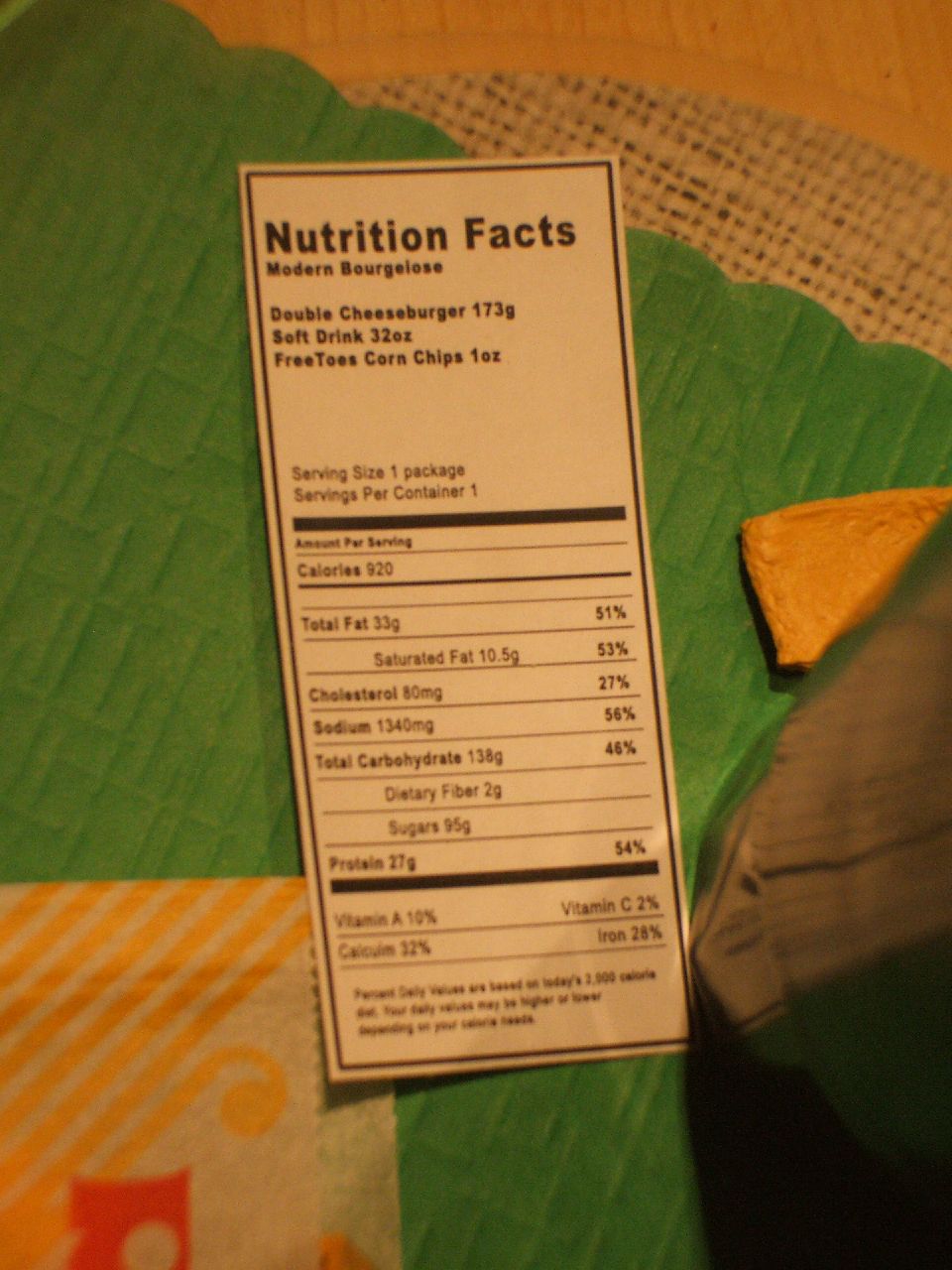The image features a detailed nutritional facts label for a double cheeseburger weighing 173 grams, accompanied by a 32-ounce soft drink and an indication of complimentary tortilla chips. The label is white with black text and black lines, meticulously outlining the nutritional content of the food items. This label is positioned on a green cloth or blanket, adding a touch of vibrancy to the background. In the upper right corner of the image, there is a beige, wicker-style basket partially visible, adding an element of texture to the scene.